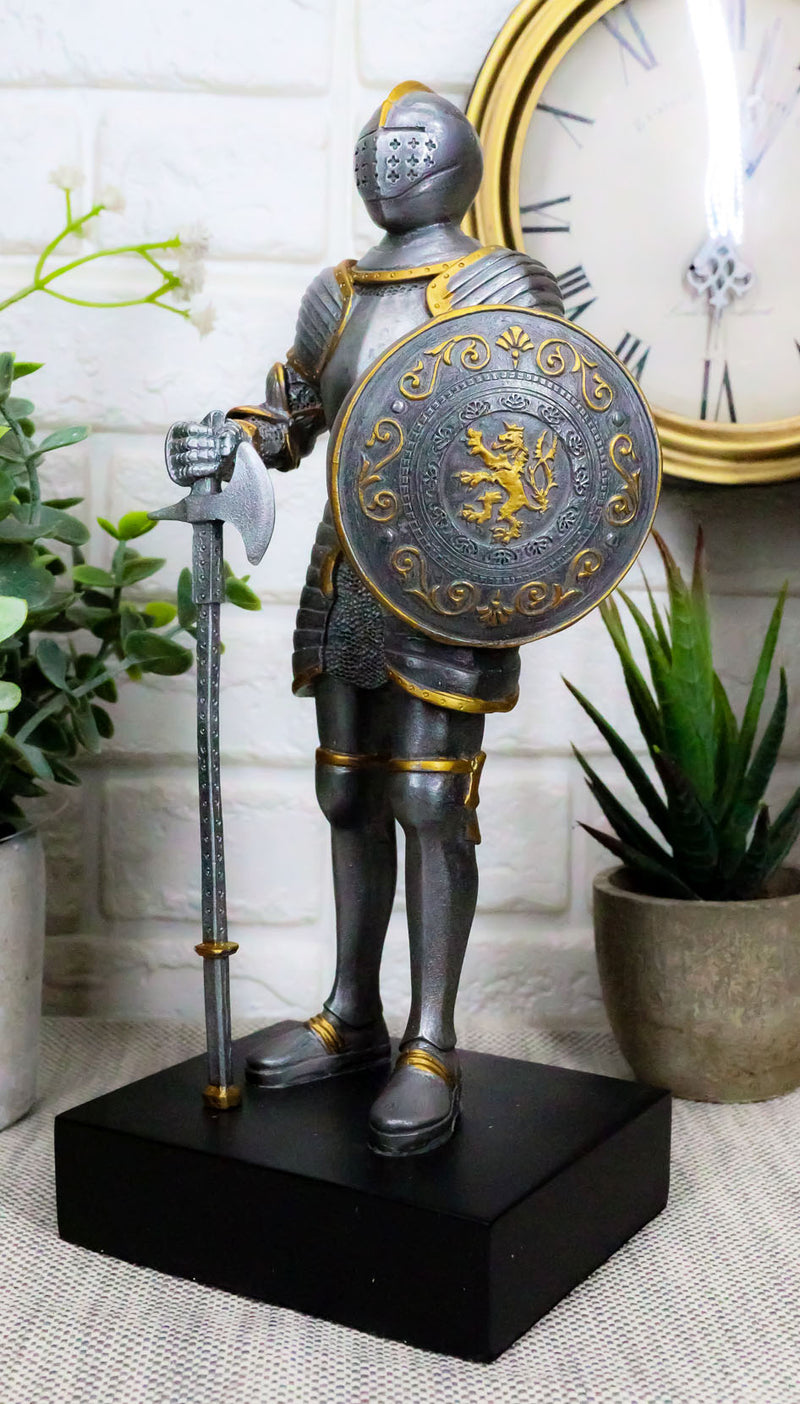The image depicts a highly detailed miniature knight figure dressed in a suit of ornate armor, positioned on a substantial black, square-shaped stand. The knight is portrayed holding an axe in his right hand and a round shield in his left. Both his armor and weapons are adorned with gold accents, with the shield uniquely featuring a central gold line. Flanking the figure are green plants in small clay pots, positioned to the left and slightly behind the knight. The scene is set against a white brick wall, which is complemented by a gold-edged round clock hanging on it. The base where the figure stands appears to be covered with a grid-patterned cloth with visible holes. Notably, the knight grips the axe by its handle, accentuating the detailed craftsmanship of the miniature.